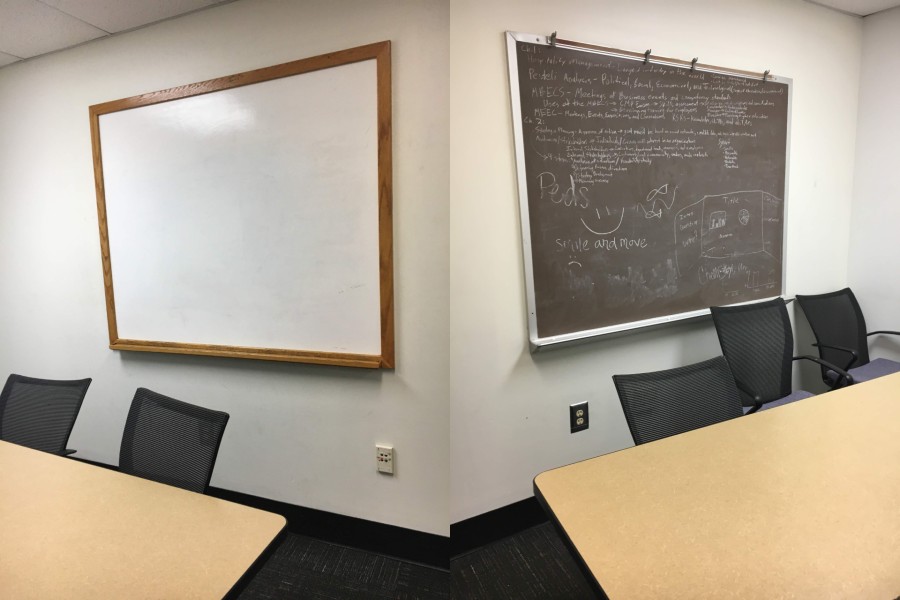The image depicts a well-lit meeting room or classroom, centered around the corner where two walls converge. On the right wall, there is a green chalkboard with detailed chalk writings, including a smiley face and the letters "P-E-D-S." The chalkboard is framed in silver trim and mounted on a white wall. Directly beneath it, there is a silver electrical outlet. In front of the chalkboard are three black chairs and a long, light brown table.

On the left wall, there is a whiteboard with a brown wooden frame, also positioned on a white wall. Below this whiteboard, there is a white electrical outlet. In front of the whiteboard are two black chairs and another matching light brown table. The room is furnished with modern black chairs and features two brown tables, ideal for meetings or collaborative sessions. The concise and functional setup is designed to facilitate both teaching and discussions, with convenient access to electrical outlets on both sides.